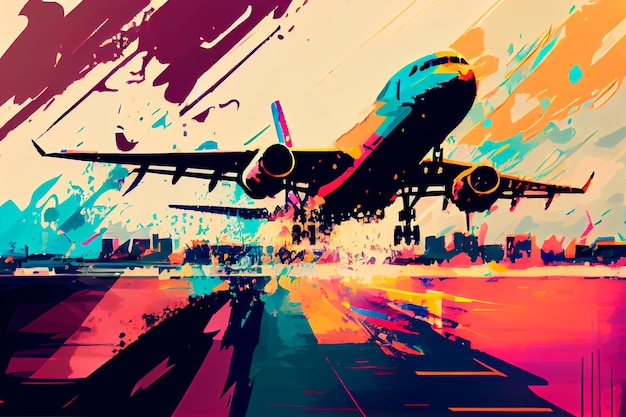The image depicts a watercolor painting with a retro aesthetic, characterized by its vivid neon colors and dynamic composition. Central to the artwork is a plane, captured in the moment of takeoff, with its nose painted in green and yellow, while the rest of its body showcases a blend of orange, yellow, pink, blue, and other vibrant hues. The plane's black underside and the pink coloration beneath the wings emphasize its powerful ascent. Jet engines are visible on both sides of the wings. The runway below the plane features a dark teal and orange palette, framed by pink ground edges, leading to indistinct city buildings in the distance. The sky above is a light peach with expressive streaks in raspberry, orange, and green, further enhancing the painting's dynamic and retro feel.